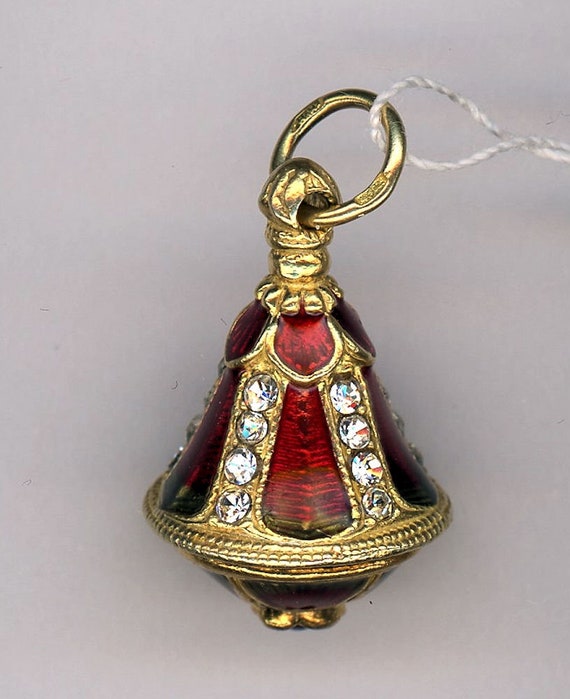This image showcases a highly detailed and ornate bell-shaped pendant, which likely serves as both a piece of jewelry and an ornament. The pendant is predominantly crafted from gold, featuring intricate filigree along its rounded base. The sides of the pendant are adorned with strips of four diamonds, each strip separated by substantial red gems that appear to be rubies. These rubies are presented in clusters at the top with individual drops extending down the sides. The top of the pendant has a gold loop, designed to be attached to a necklace, and is threaded with a piece of twisted fiber string, which might be a price tag holder. The entire piece exudes an elegant, festive charm, reminiscent of a fancy Christmas ornament. The photograph captures the pendant against a plain white background, emphasizing its intricate details and sparkling features.